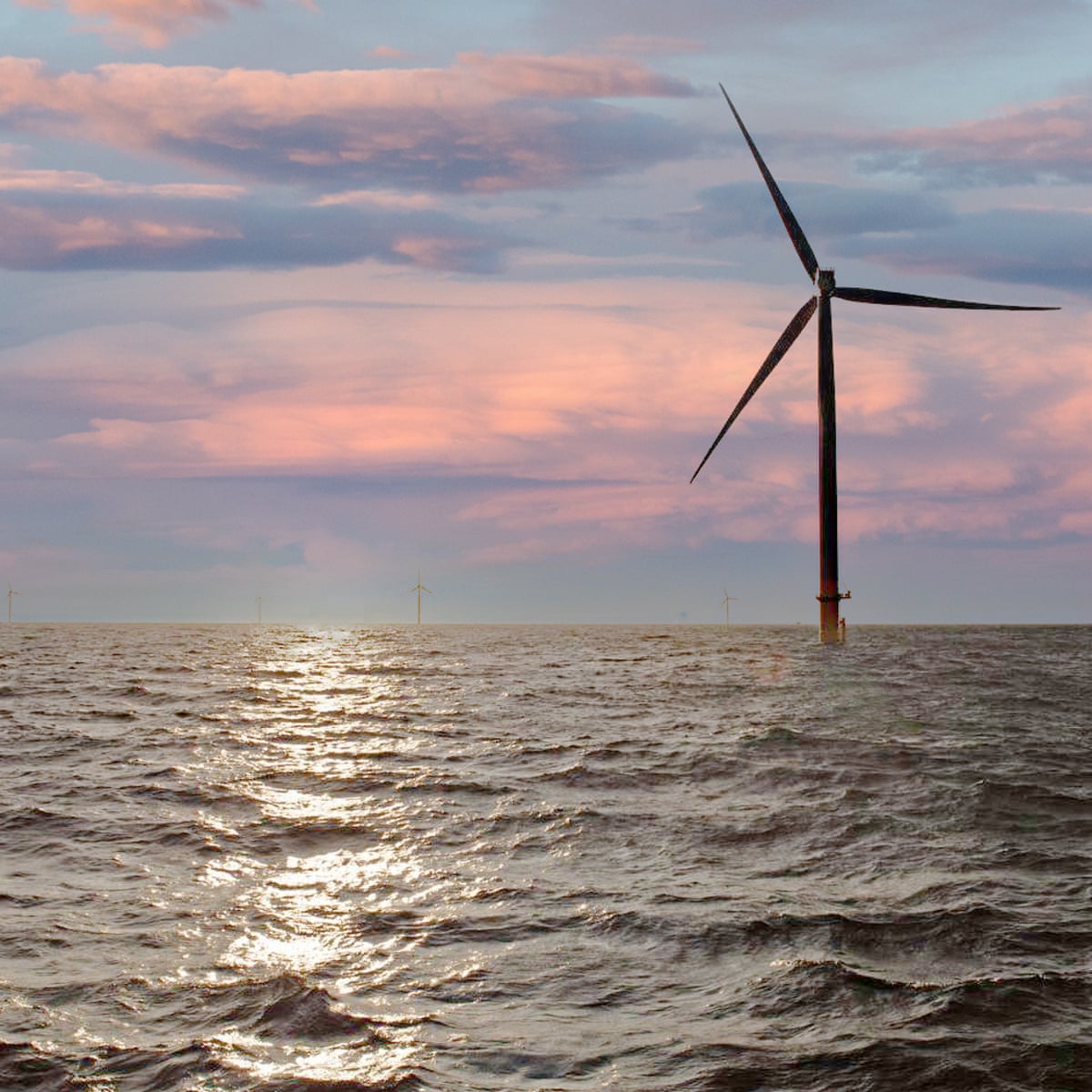The image depicts a tranquil ocean scene during either the early morning or late evening. The expansive body of dark navy greenish-blue water fills the bottom half of the image, with gentle waves that catch the reflection of the sun, creating a shimmering path from the lower left to the center. Dominating the middle right portion of the image, a large, tall windmill rises from the water, featuring three blades that likely extend 10 feet each. This windmill appears dark brown to black with hints of red. Further in the distance, at the horizon line in the center, are faint silhouettes of four more windmills, barely distinguishable. The upper half of the image showcases a picturesque sky resembling cotton candy with hues of light blue, pink, purple, and white clouds, suggesting a serene time of day transitioning between daylight and dusk. There is no land in sight, indicating this scene is set far out in the ocean.